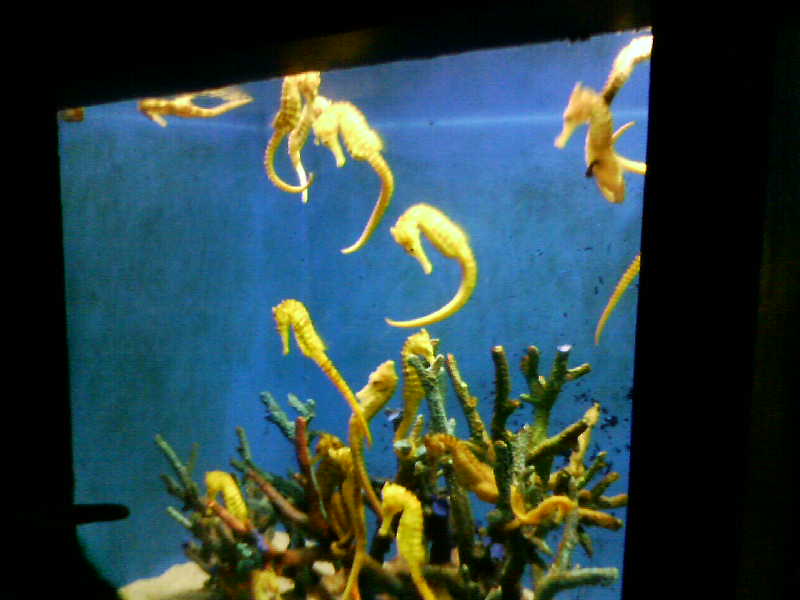This image depicts an aquarium exhibit showcasing numerous yellow-gold seahorses, set against a vivid blue backdrop inside the tank. The tank is brightly illuminated, casting the seahorses into clear view while the surrounding environment remains almost pitch black. The aquarium appears crowded, with seahorses entangled in branches or possibly fake coral at the bottom, and others floating above. A few seahorses are positioned at varying heights, including one at the very top that may be deceased. The seahorses have a toy-like appearance, adding to the surreal quality of the scene. The green and yellow coral in the middle further enhances the exhibit's colorful aquatic theme.